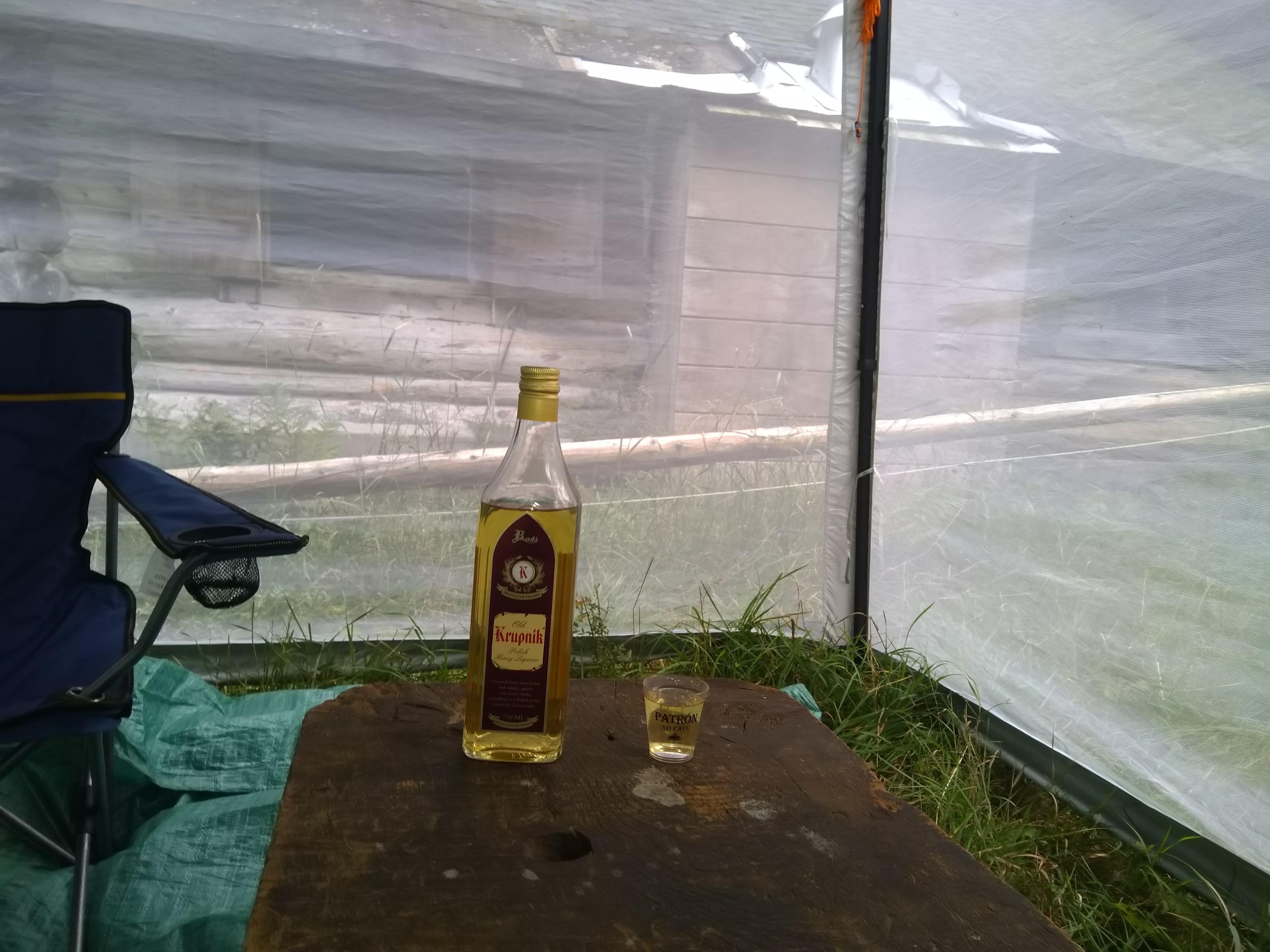In a cozy yet rustic outdoor setup, a coarse wooden table, showing signs of wear and disrepair, supports a bottle of Krupnik, a yellowish liquor, and a matching shot glass labeled Patron. The scene unfolds inside a see-through plastic mosquito tent, pitched over an area with some overgrown grass peeking through the gaps. To the left, a dark blue canvas foldable camping chair with a mesh cup holder is positioned on top of a teal tarp. In the background, a worn wooden house with weathered shutters and damaged roofing stands visible through the transparent tent walls. The overall ambiance suggests a relaxed, perhaps slightly weathered, outdoor get-together with elements of both nature and human warmth blending seamlessly.